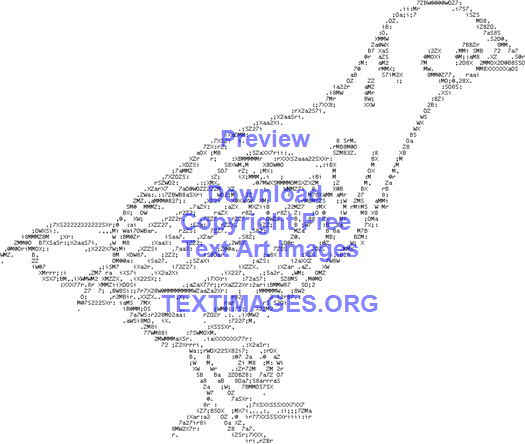The image features an intricate ASCII art rendering of a bird, reminiscent of 1980s laser dot printing. Composed of various small black characters and numbers, the bird is depicted in a side profile with one leg lifted and the other firmly on the ground. Its tail is distinctly visible, and it appears to be gazing away from the viewer. The bird's wing is also discernible among the lines of text. Overlaying this detailed bird outline is blue text that reads "Preview" at the top, followed by "Download," "Copyright Free," "TextArtImages," and at the bottom, "TextImages.org." The background is predominantly white, allowing the meticulous composition of characters to form the bird’s elegant shape.